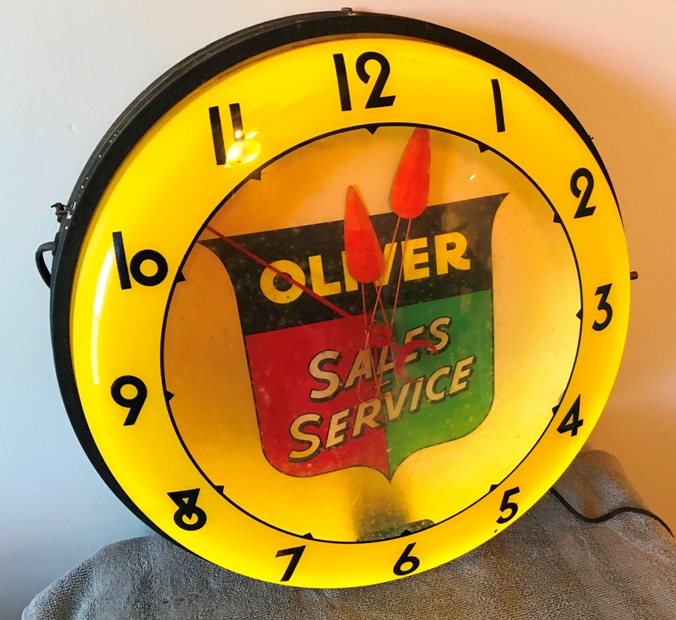The image depicts a watch placed on a gray microfiber cloth that serves as the ground, accentuated by black edges. The background is a plain white, providing a stark contrast to the subject. The watch's body is predominantly black, with vibrant yellow accents encircling the perimeter. The hour hand is positioned vertically, pointing upwards, while the minute hand is angled slightly past the hour, and the second hand rests between the 10 and 11 o'clock marks. At the center of the watch face is a shield emblem; its upper section is black, the bottom left segment is red, and the bottom right segment is green. The center of the shield features an inscription that seems to read "author, self-service," suggesting a personalized or customized design.